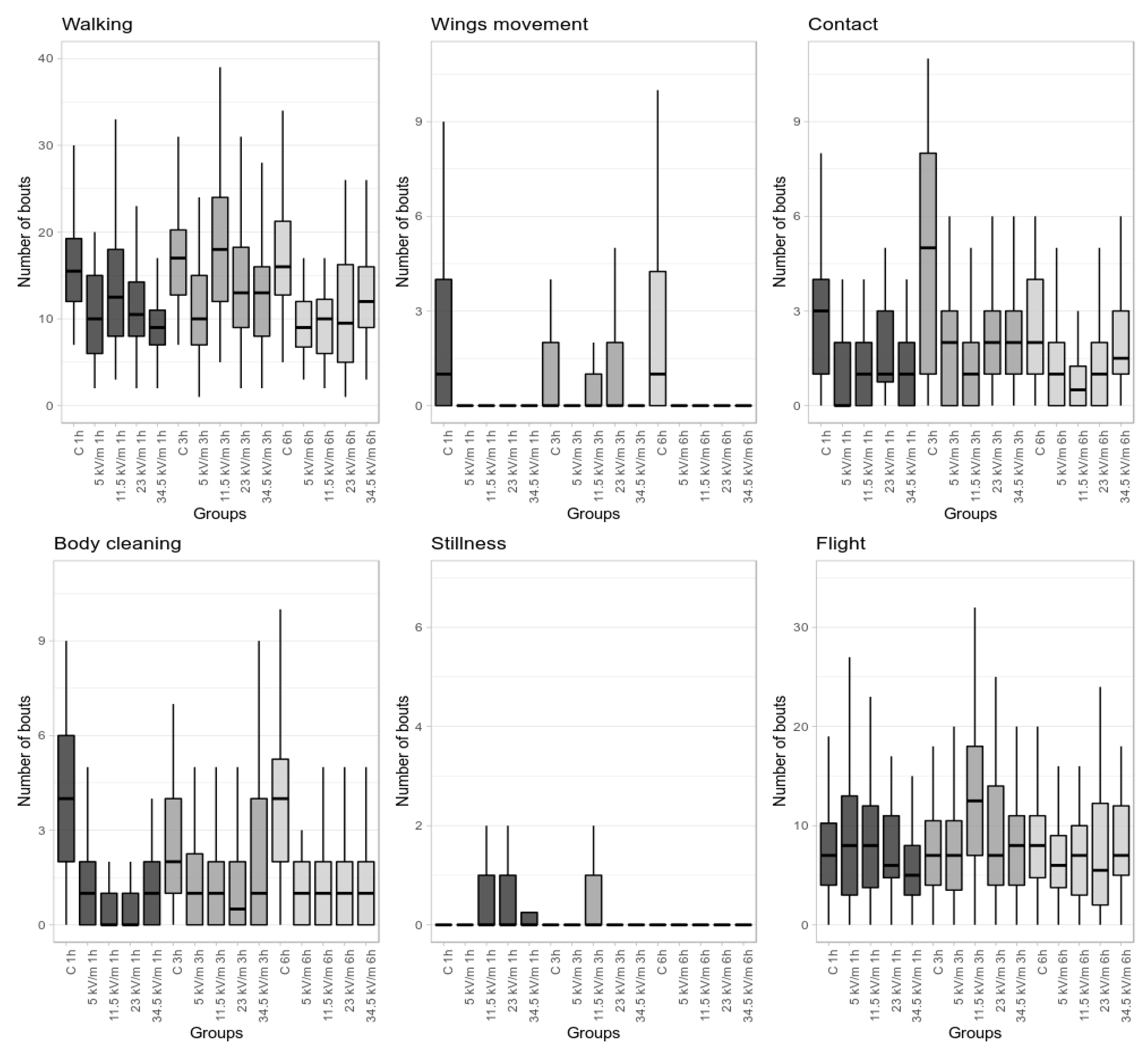The image showcases six distinct bar charts labeled as walking, wing movement, contact, body cleaning, stillness, and flight. Each chart uses the vertical axis to represent the number of bouts, while the horizontal axis likely tracks groups or categories labeled in kilovolts per meter (KV/m). The charts exhibit varying amounts of data points; walking, contact, body cleaning, and flight appear more populated, whereas wing movement and stillness contain fewer points. The overall theme of the charts seems to be related to some form of behavioral or medical research, although specific details about the heading or exact measurements are not provided due to their small and challenging-to-decipher size. The graphs are rendered in black, white, and gray, with a clear emphasis on tracking bouts of different behaviors over a standardized metric.